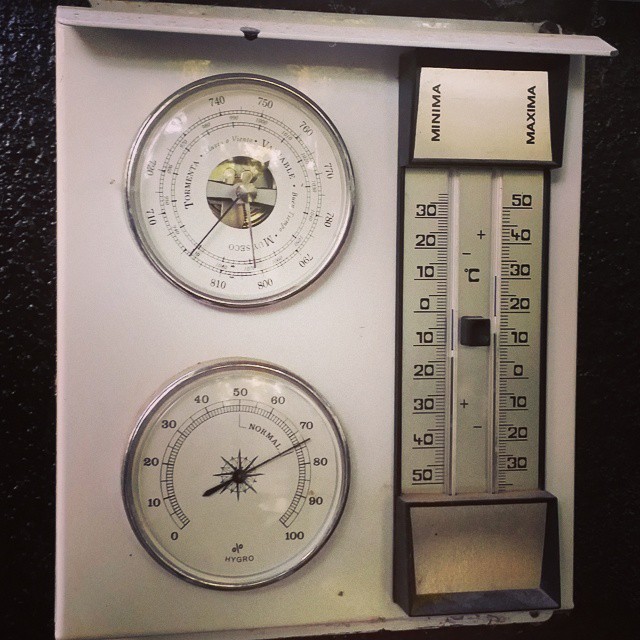The photograph captures a vintage thermometer and hygrometer setup mounted against a black wall. The primary structure is a large rectangular unit featuring a white metal shelf-like piece at the top. On the left side of the rectangle, there are two circular dials. The upper dial, encircled by a metal band, has a white face with two clock-like hands. This appears to be a thermometer with the brand or model name "TYMENTA" visible. The dial’s perimeter is marked with numbers which may represent distances or units.

Below it, the second circular dial, bordered by a silver band, features a black hand and is labeled "HYGRO" at the bottom. This hygrometer dial is numbered from 0 to 100 in 10-unit increments, moving clockwise.

To the right of the dials, a long, rectangular thermometer display is segmented into two vertical columns labeled "minima" and "maxima." The first column is marked with numbers descending in the order of 30, 20, 10, 0, -10, -20, -30, -40, -50. The second column shows a descending sequence of 50, 40, 30, 20, 10, 0, -10, -20, -30, -40. This detailed instrumentation likely serves to measure and display both temperature and humidity with precision.